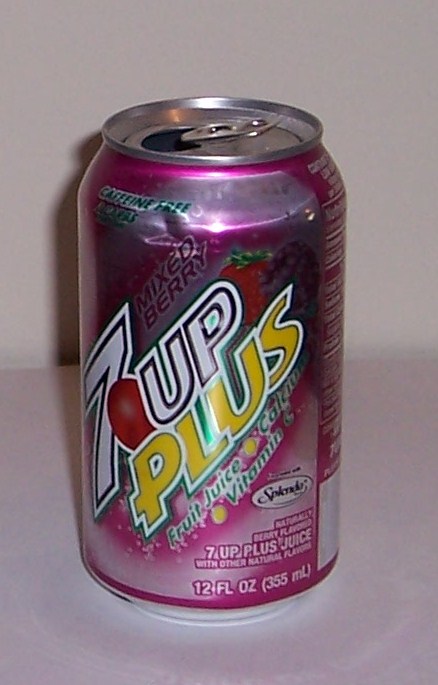In this detailed image, we see a can of 7up Plus soda with a mixed berry flavor prominently displayed on a table with a white surface. The can features a vibrant blend of purple and pink hues. The iconic 7up logo is easily recognizable with a large white "7," a red dot, and "up" in white text. Below this, "PLUS" is spelled out in bold, capital yellow letters with a white outline.

A picture of a strawberry suggests the mixed berry flavor, enhancing the fruity appeal. Beneath "PLUS," additional benefits are highlighted in smaller, greenish font with white outlines, listing "fruit juice," "calcium," and "vitamin C." The Splenda logo indicates the presence of the artificial sweetener. The can holds 12 fluid ounces of the beverage, and the right-hand side starts to reveal the nutritional facts, offering a glimpse into the product's dietary information.